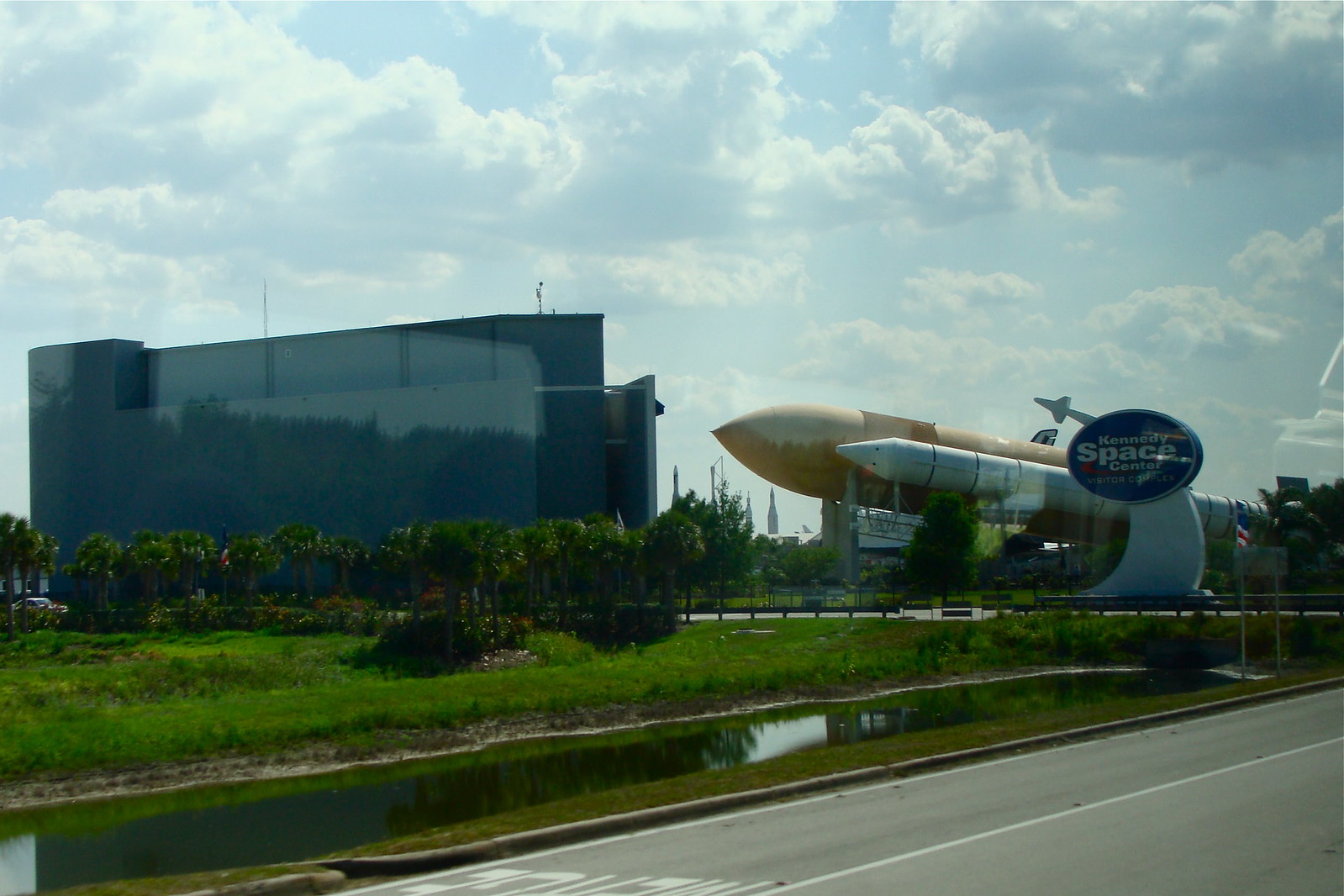The photograph captures a sunny day at the Kennedy Space Center visitor area. The sky is a vibrant blue, dotted with fluffy white clouds. Dominating the center of the image is a sleek, reflective blue building. To its right stands a makeshift space shuttle composed of two large rockets: one gold with a pointed tip and another white, resembling a crayon. A prominent blue sign with "Kennedy Space Center" written in white text on a white stand is positioned near the rockets. In the foreground, lush green grass and small shrubbery frame a murky creek of water that runs parallel to a gray roadway visible at the lower edge of the photo. Palmtrees and other short, bushy-topped trees are scattered in front of the building, enhancing the natural beauty of the scene.